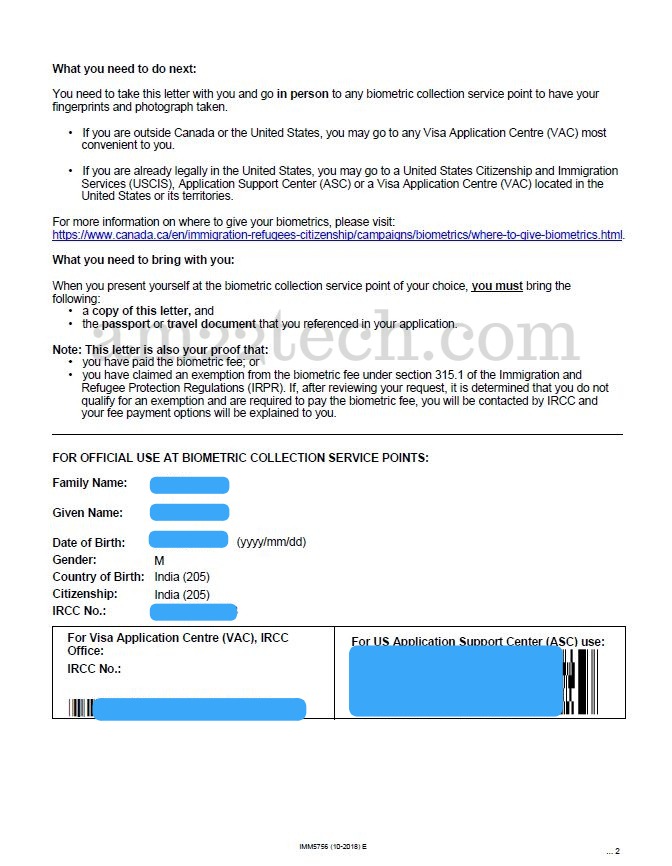This image features an official document with a predominantly white background, filled with text and various sections formatted for collecting biometric data. 

**Header Section:**
- At the very top, the document is titled with instructions: "What do you need to do next?"
- It outlines that the recipient must bring this letter in person to any biometric collection service point to have their fingerprints and photograph taken. Specific locations include a visa application center (VAC) for those outside Canada or the U.S., or a U.S. Citizen Immigration Services (USCIS) Application Support Center (ASC) or a VAC within the U.S. or its territories.

**Body Section:**
- The main section below the instructions lists several fields, including Family Name, Given Name, Date of Birth, Gender (notated as 'M' for Male), Country of Birth (India), Citizenship (India), and RICC Number.
- Many of these fields have blue sections blocking out crucial information for privacy, particularly the Family Name and Given Name fields.

**Footer Section:**
- At the bottom of the document, there are additional sections labeled for specific use cases:
  - "For official use at biometric collection service points."
  - "For Visa Application Center (VAC) use."
  - "For RICC office use," along with an obscured barcode covered by a blue section.
  - "For U.S. Application Support Center (ASC) use," accompanied by another obscured barcode with a blue overlay.

**Miscellaneous:**
- The page also contains links and further instructions on what to bring to the biometric appointment.
- A faint "am22tech.com" logo appears in gray on the document, indicating the source of the form or information.

Overall, this document appears to be a formal letter instructing the recipient on the next steps for their biometric data collection, necessary for immigration or visa purposes.